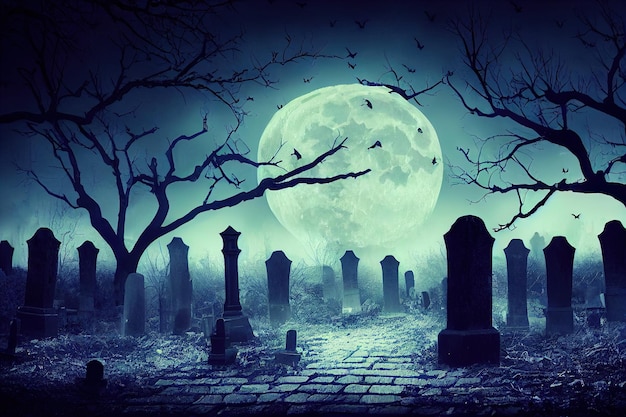The image depicts an eerie night in a graveyard characterized by an expansive full moon that dominates the background, casting an ethereal glow over the scene. The moon, which takes up a significant portion of the sky, illuminates the graveyard's cobblestone floor and the numerous gravestones scattered throughout. The scene is marked by stark, leafless trees on either side, their barren branches reaching out like skeletal arms. Between these trees, several birds or bats flutter, their forms silhouetted against the moonlit sky, enhancing the ominous atmosphere.

The graveyard appears deserted and neglected, with signs of overgrown shrubs and debris adding to the spooky ambiance. There are around 11 gravestones of varying sizes; one notable tombstone is particularly wide, contrasting with the many narrower ones. The entire scene is suffused with dark hues of gray, blue, and purple, creating a chilling, Halloween-esque aesthetic. Given the artistic style, the image appears to be either a detailed drawing or a digital rendering rather than a photograph, making it an ideal depiction for a spooky Halloween setting.